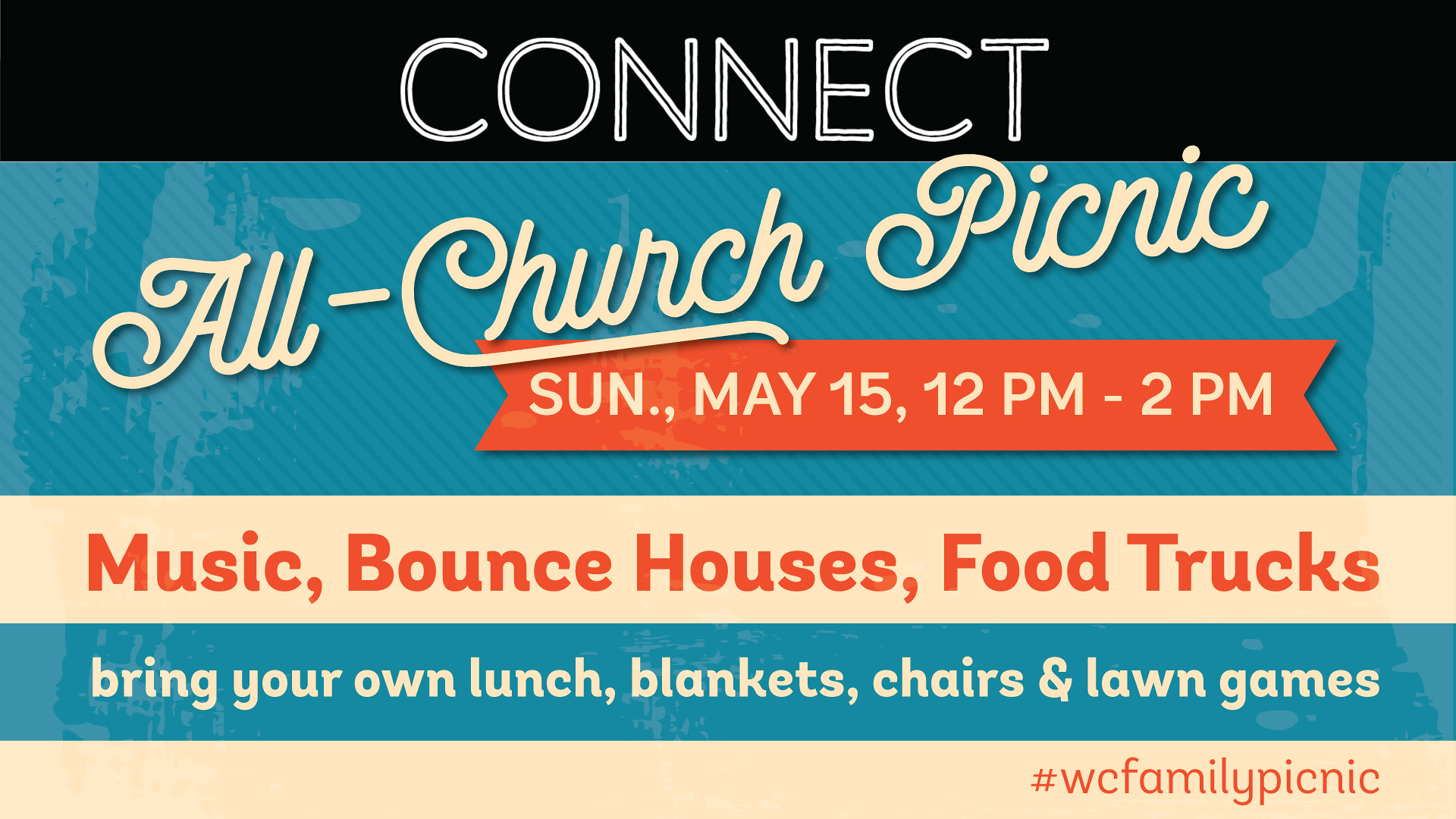This vibrant electronic advertisement promotes an all-church picnic with a color scheme of black, blue, peach, and cream, featuring white, orange, and red lettering. At the top of the ad, "Connect" is prominently displayed in white text against a black background. Below, "All Church Picnic" is elegantly written in peach cursive on a blue backdrop, followed by event details: "Sunday, May 15th, 12pm-2pm" in contrasting red text. The advertisement highlights activities such as music, bounce houses, and food trucks, listed in peach text within a cream-colored box. Further instructions encourage attendees to bring their own lunches, blankets, chairs, and lawn games, again in peach text on a blue background. The event's hashtag, #WCFamilyPicnic, is neatly placed in red text on the bottom right, tying the design together.